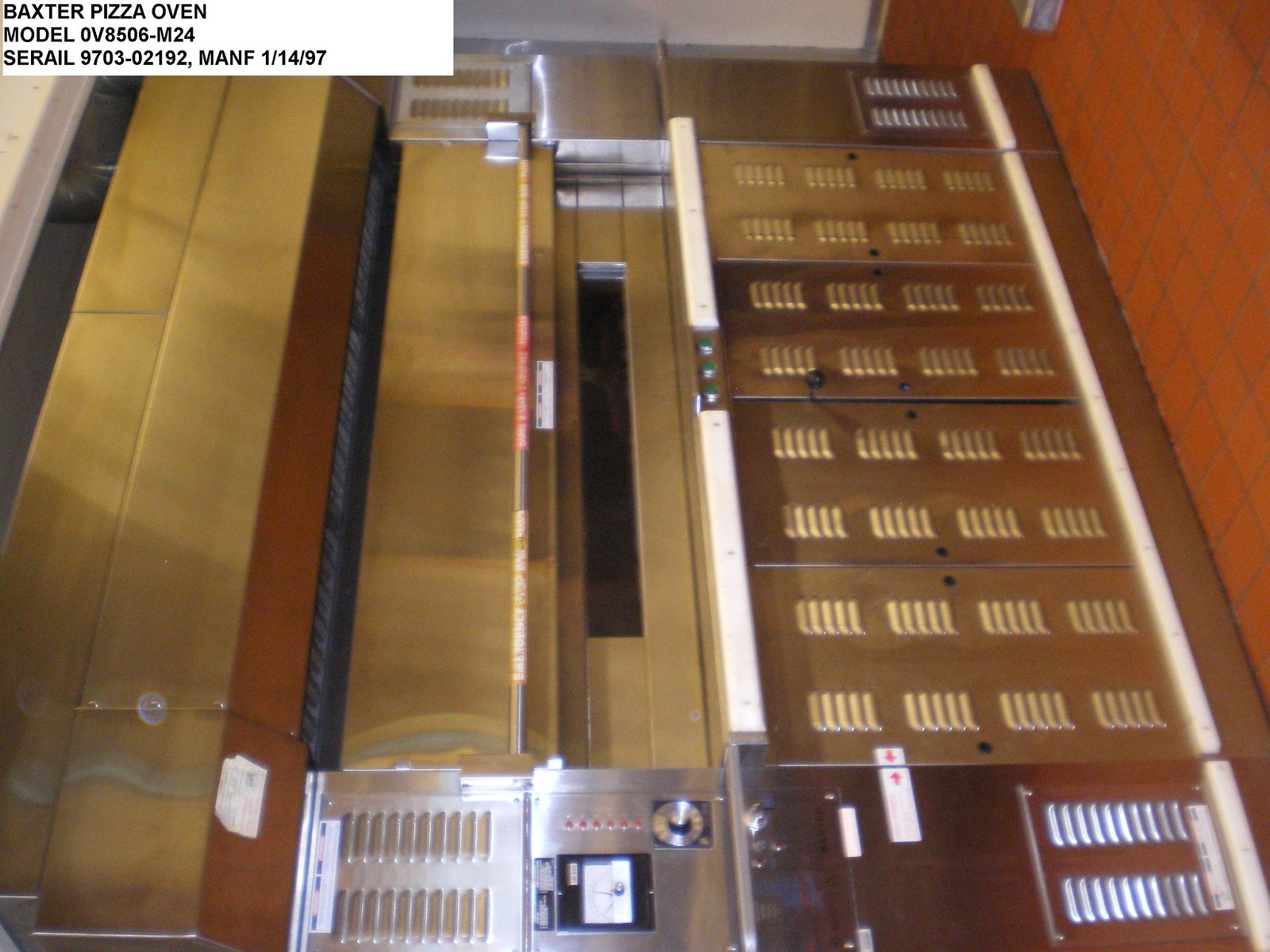The image depicts a large, industrial Baxter Pizza Oven, Model OV8506-M24, situated against an orange tile wall. The stainless steel appliance appears sideways due to the photograph's orientation, giving the impression that the oven is vertical. The top left corner features a text label, providing the model number, serial number 9703-02192, and the manufacturing date, January 14, 1997. The pizza oven showcases rows of vents and a sizable drawer-like opening where pizzas are inserted. Despite some confusion caused by the rotated image, the oven's silver and gold components, along with its grates and control panel, are distinctly visible, conveying the heavy-duty nature of this pizzeria staple.